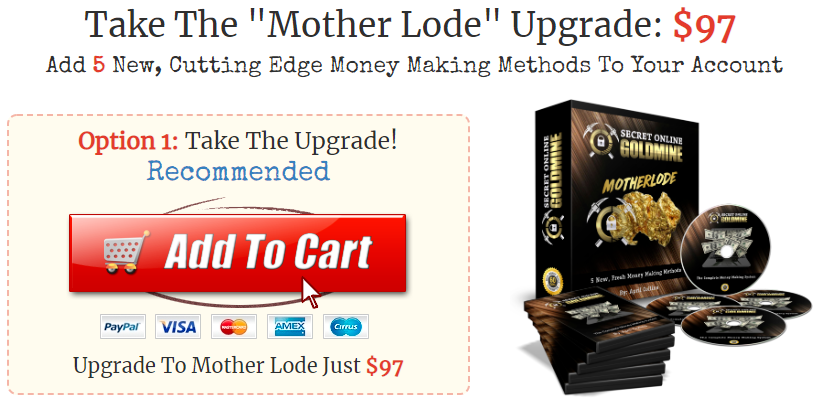This image depicts a detailed product advertisement for an online money-making program called "Motherlode." The advertisement has a clean white background with prominent black text at the top, stating: "Take the Motherload Upgrade" in quotes. Below this, in red text, it indicates a price: "$97". The primary message continues with the offer to "add five new cutting-edge money-making methods to your account," with the number "five" highlighted in red.

On the left side of the image, within a dotted red line square, there is an option labeled "Option 1: Take the Upgrade!" The word "recommended" is prominently displayed in blue beneath this option. A striking red rectangular button, labeled "Add to Cart" in white letters, features an accompanying shopping cart icon. Adjacent to the button, a mouse cursor hovers over various payment options, including PayPal, Visa, MasterCard, Amex, and Cirrus.

On the right side of the image, there is a visual representation of the product packaging. The packaging appears as a black case adorned with white and gold text that reads "Secret Online Gold Mine Motherlode." The case features images of gold nuggets and pickaxes, evoking a mining theme. Next to it, there are stacks of CD-ROMs and DVDs, suggesting a comprehensive set of physical media accompanies the program. The entire visual presentation aims to entice viewers to upgrade their purchase for $97 to gain access to advanced money-making strategies.